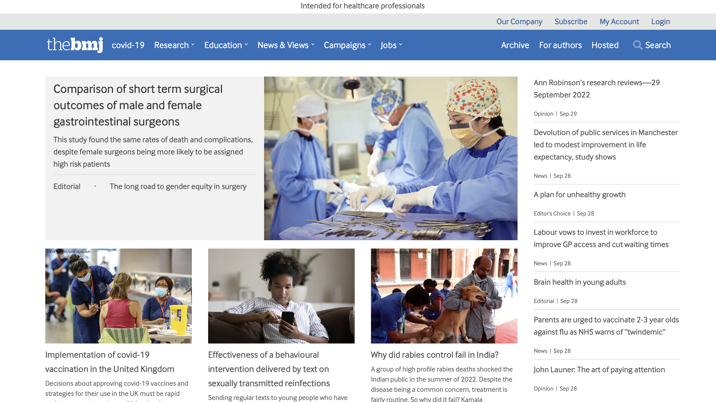**Title: The BMJ - COVID-19 Research**

The webpage of The BMJ, an esteemed medical journal for healthcare professionals, prominently displays comprehensive resources, including sections for COVID-19 Research, Education, News and Views, Campaigns, Jobs, Archive for Authors, and a Search feature. At the center of the page, an image shows three medical professionals dressed in blue gowns, scrub caps, gloves, and face coverings, engaged with various medical tools.

On the far right column is a series of headlines, including:
- "Anne Robinson's Research Reviews, 29 September 2022"
- "Devolution of Public Services in Manchester Led to Modest Improvement in Life Expectancy, Study Shows"
- "A Plan for Unhealthy Growth"
- "Labour Vows to Invest in Workforce to Improve GP Access and Cut Waiting Times"
- "Brain Health in Young Adults"

Additional imagery on the page includes:
- To the far left, a healthcare professional (possibly a nurse or doctor) administering an injection to a woman's arm.
- An individual sitting and looking down at a cell phone, accompanied by the caption: "Effectiveness of a Behavioral Intervention Delivered by Text on Sexually Transmitted Reinfections."
- On the far right, a man standing next to a dog, holding it gently around the neck, with the caption: "Why Did Rabies Control Fail in India? A Group of High Profile Rabies Deaths Shocked the Indian Public in the Summer of 2022."

Together, these elements paint a vivid picture of an informative and engaging web resource for those in the medical field.